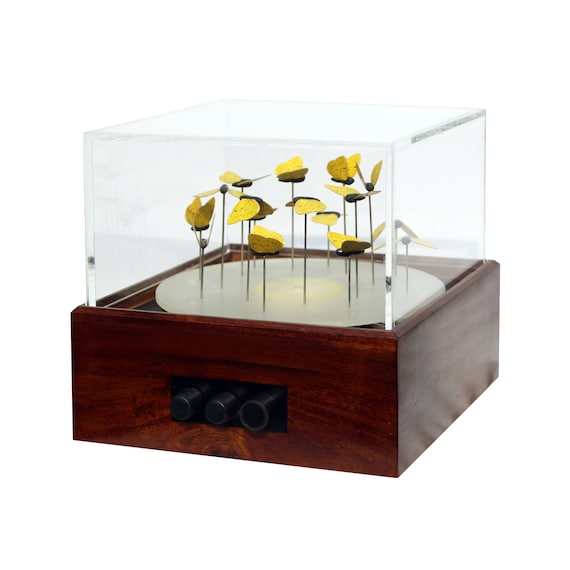The image depicts a cubicle-shaped box with a dark brown, almost cherry wood-like base featuring horizontal grains on the front. There are three cylindrical, black knobs arranged in a horizontal row on the front. The lid is transparent, possibly made of glass or plastic, fitting snugly atop the wooden base. On a solid white background with no text or border, the focus inside the box is a light gray circular platform. Emanating from it are numerous thin, needle-like stems, dark brown or dark gold in color, each topped with what appears to be a yellow butterfly with delicate wings and a dark brown body. The butterflies are mounted at varying heights, creating a visually intriguing composition of fluttering yellow forms.